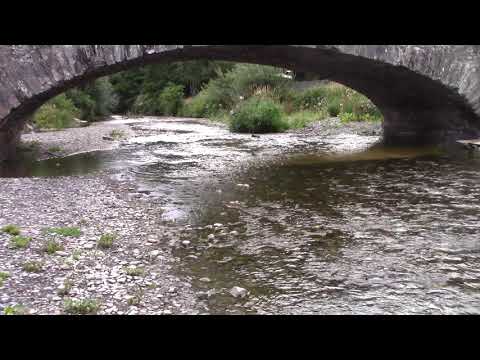The image features a picturesque river scene dominated by lush greenery and vivid natural elements. In the foreground, the river, with its greenish-gray, shallow waters, meanders from the bottom right to the center of the image. The left bank of the river is lined with a variety of small stones and patches of green grass emerging from the gravel. Contrasting textures and colors, such as the dark brown of the bridge and various shades of green from the surrounding flora, contribute to the image's vibrant palette.

Toward the top of the image, partially obscured by the framing, is a rustic wooden arched bridge. Only the lower part of this bridge is visible, indicating its distinct arch shape made of dark brown bricks or wood. The scene is framed by an abundance of verdant greenery, with tall trees and dense bushes on either side of the river. The setting exudes a peaceful, outdoor ambiance, likely captured in the middle of the day, emphasizing the serene interaction between the natural elements and the gently flowing stream beneath the bridge.